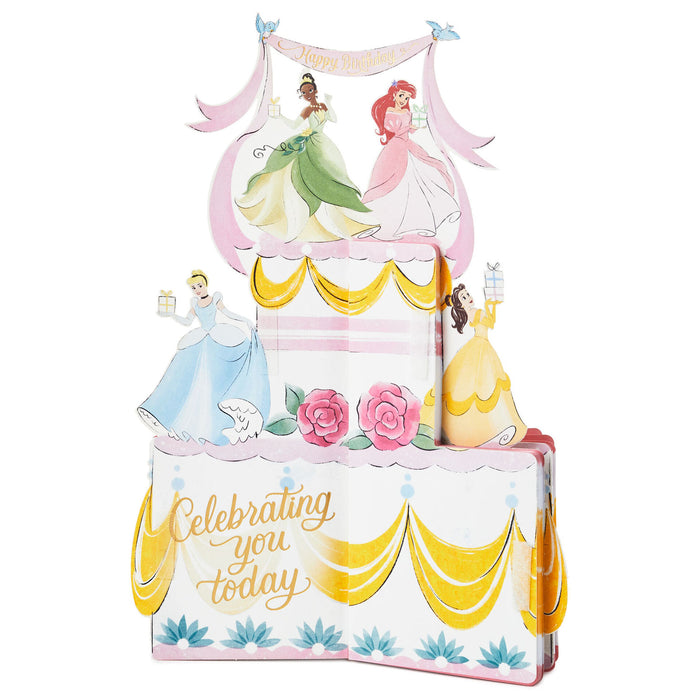An image depicts a detailed table decoration designed for a little girl's birthday celebration, themed around Disney princesses. The decoration is likely made of cardboard and features a tiered cake design with delicate accents. At the top, a ribbon held by little bluebirds reads "Happy Birthday." Below, Princess Tiana and Ariel stand beneath this banner, each holding a gift. Cinderella, in a blue dress, and Belle, in a yellow dress, are positioned on either side of the cake, also holding presents. The decoration includes vibrant elements such as pink and blue flowers, a yellow border, and pink lace cascading from the top. At the base of the decoration, the phrase "Celebrating You Today" is prominently written in gold, complemented by gold ribbons and pink flowers.